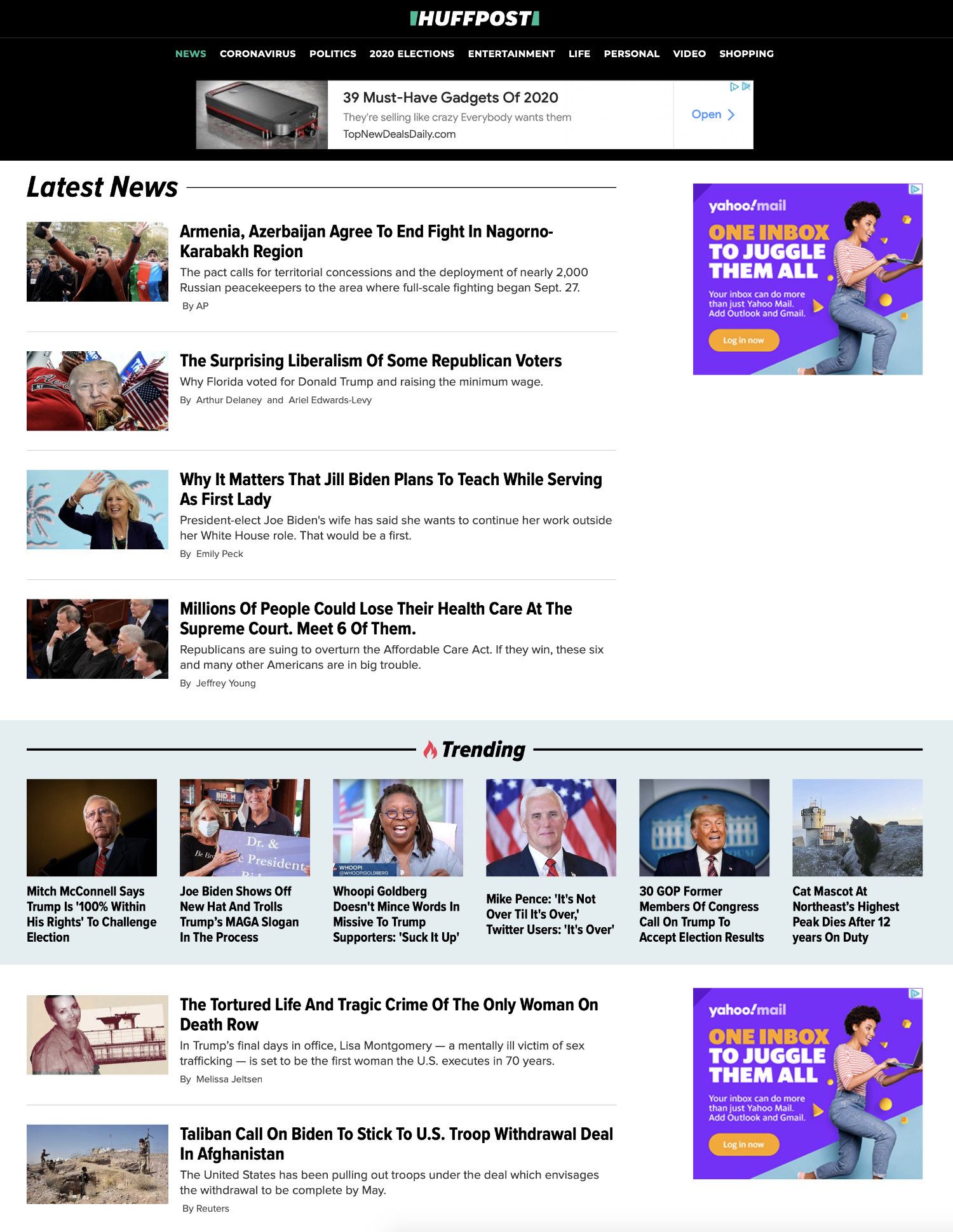This screenshot captures the layout of the HuffPost website. At the top center of the page, the HuffPost logo is prominently displayed. A black navigation bar runs across the top of the page, featuring a menu and an advertisement. The menu is centrally aligned and includes the following categories: News, Coronavirus, Politics, 2020 Elections, Entertainment, Life, Personal, Video, and Shopping. The advertisement, hosted by topnewsdaily.com, is positioned alongside this menu.

Below this bar, the section labeled "Latest News" showcases four articles listed in vertical succession. The first article headline reads, "Armenia Agreed to End Fight." The second article discusses, "The Surprising Liberalism of Some Republican Voters." The third article is titled, "Why It Matters That Joe Biden Plans to Teach While Serving as First Lady." The fourth and final article highlights a critical issue: "Millions of People Could Lose Their Health Care at the Supreme Court; Meet Six of Them."